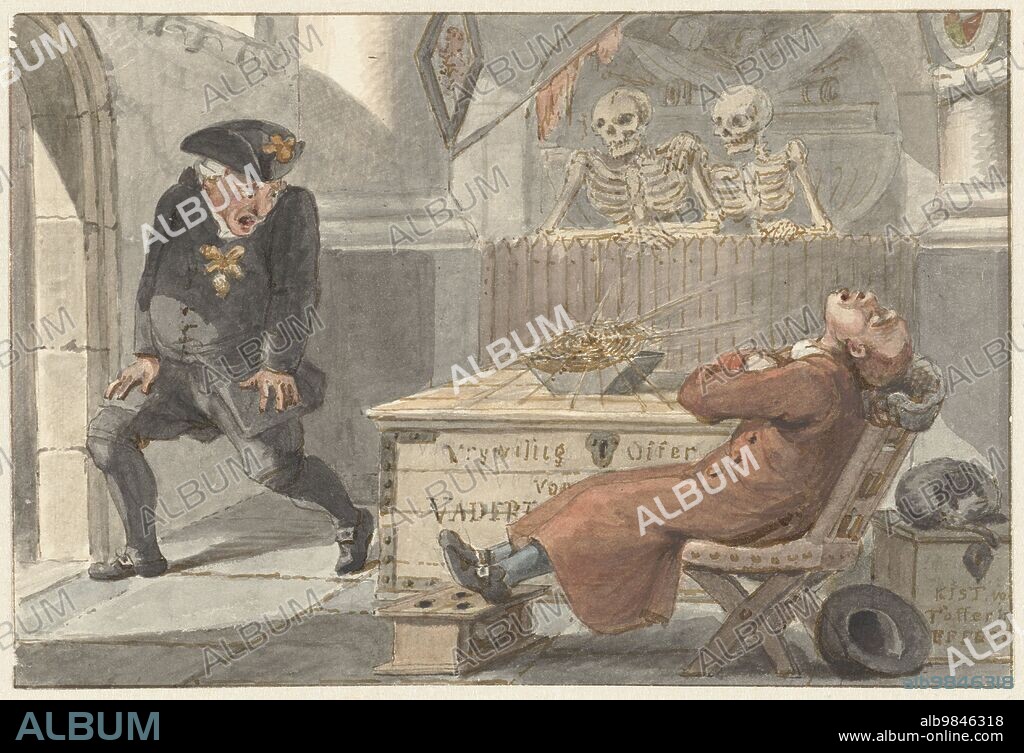The image is a vividly detailed painting featuring a striking encounter between two men and two skeletons, laden with atmospheric tension. In the foreground, a man clad entirely in black—complete with a triangular hat, black shirt, and black pants—stands with eyes wide open and mouth agape, gazing down with a shocked and almost fearful expression. Opposite him, a second man is seated on a chair, slumped back with his head tilted upwards, seemingly asleep. He is adorned in a red cloak and an old-fashioned white wig. 

Behind them, two skeletons loom ominously, peering over a fence that separates them from the men. Their skeletal figures starkly contrast with the painting’s richly colored characters. To the side, a cat peacefully dozes on a box, adding an eerie calm to the otherwise tense scene. The background is detailed with marble columns that suggest a grand, perhaps historical, setting. A mysterious object, possibly a dish with a spider web, is also part of the composition, adding to its intricate and surreal nature.

The painting has a watermark text "A-L-B-U-M" scattered throughout, and another reference to "www.album-online.com" with the word "ALBUM" prominent in blue letters against a black border at the bottom, indicating it possibly belongs to an online collection.

This artwork fuses elements of historical attire, supernatural presence, and a blend of fear and serenity, encapsulated in a deeply engaging and mysterious scenario.